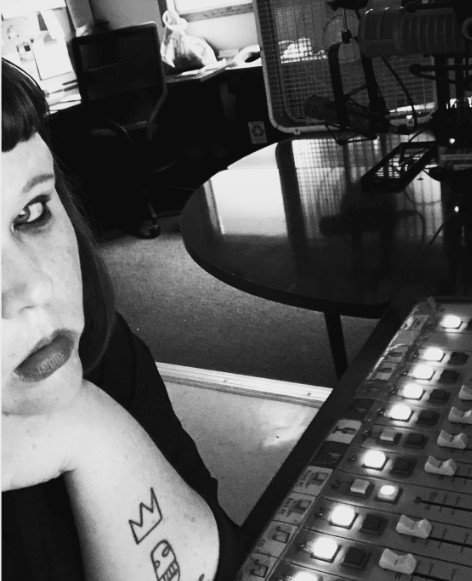This black and white photo captures an angled, partial view of a woman in an emo style, characterized by her short bob haircut with very short bangs, thick black eyeliner, and dark lipstick. She has pale skin and a distinctive tattoo on her right breast, featuring a stick figure man with teeth and a crown. Dressed in a black sweater with her cleavage exposed, she sits with an unimpressed, pouty expression in front of a lit-up soundboard, likely in a recording studio or office space. The soundboard is filled with various controls and illuminated indicators, all sliders set to zero. To her right, there is a glossy black table with a box fan and a lantern, and behind her, a corner desk with an ergonomic black mesh chair, a plastic bag, and additional office items, including a studio microphone and a lamp. The floor beneath her transitions from concrete to a gray carpet with a metal trim to hold the carpet down and separates it from the linoleum flooring in the foreground. The exposed power point on the wall and additional office furniture in the background complete the scene.